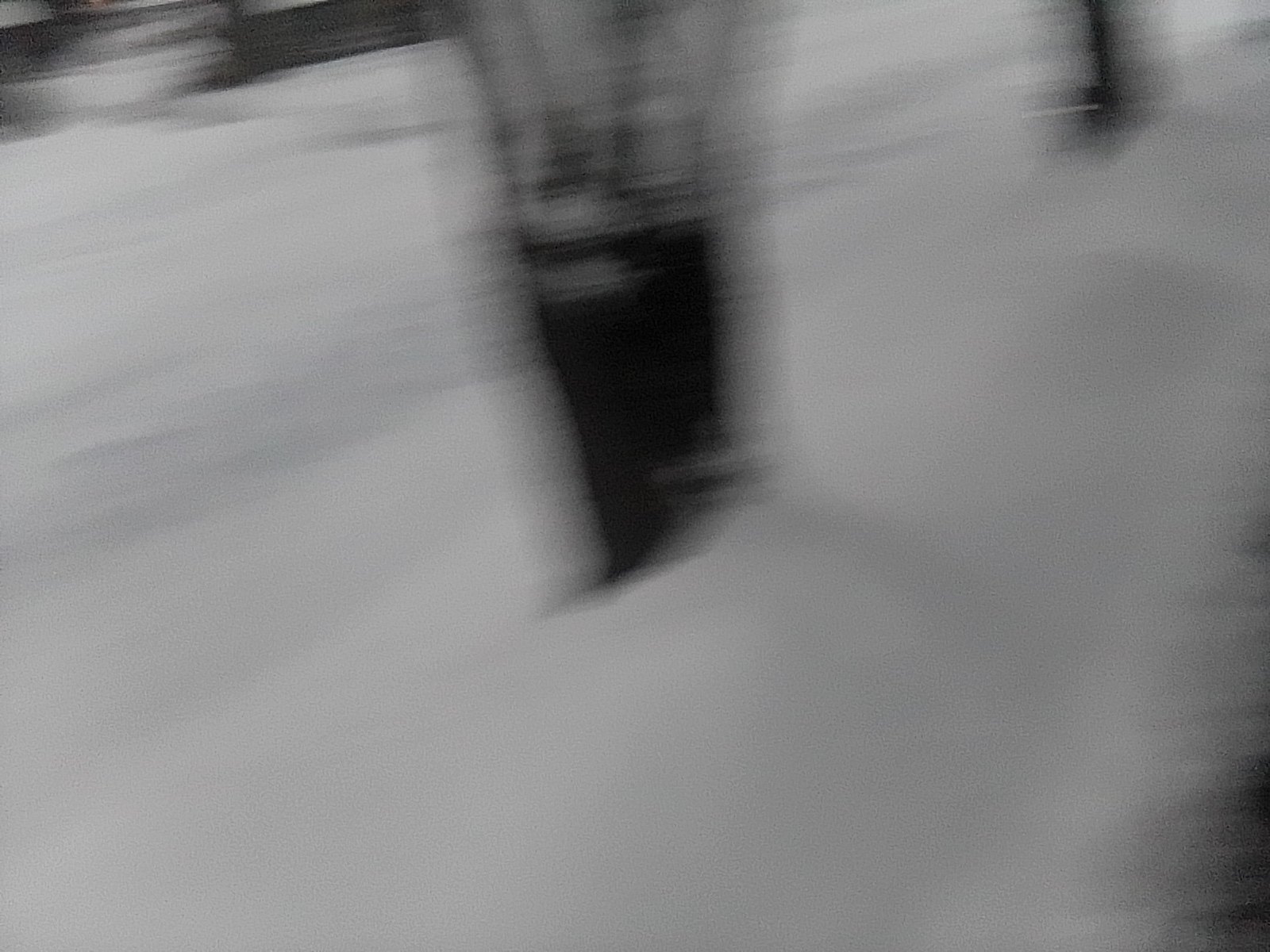This photograph is highly blurred, making the scene challenging to interpret. The image predominantly features a snowy landscape with several indistinct snowbanks. Amidst the snowbanks, there are several dark objects adorned with white text, albeit unclear due to the blur. The foreground exhibits a shaken, almost distorted effect, suggesting the camera was moved during the shot. Stray black lines are also visible throughout the image. In the distant background, faint outlines that resemble concrete steps lightly dusted with snow can be discerned. Overall, the graininess and lack of focus render it difficult to clearly define the elements within the photograph.